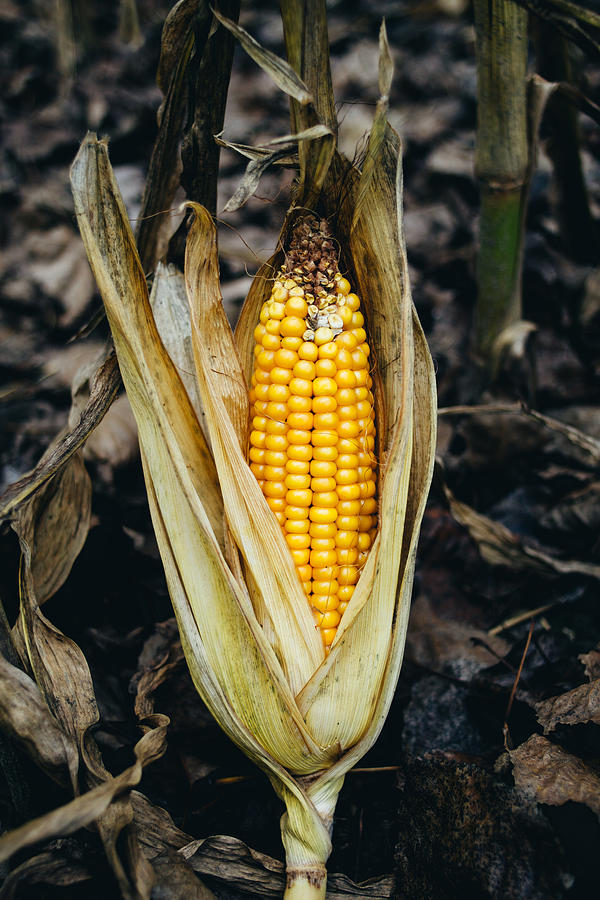The photograph depicts a vibrant ear of corn in its natural setting. The corn's bright yellow kernels are revealed as the light yellow-green husk is peeled back, though the tip of the cob shows signs of rot, marked by a transition to brown and gray-white coloration. This ear of corn is nestled among an assortment of dried, brown leaves that litter the ground, enhancing the rustic feel of the scene. Directly behind the corn, green bamboo stalks rise from the ground, adding a touch of greenery to the otherwise drab and dreary background. The image, taken outdoors possibly in the late afternoon, captures the subtle illumination of sunlight casting a gentle glow on the corn, making it the vibrant centerpiece against a shadowed, nondescript background.